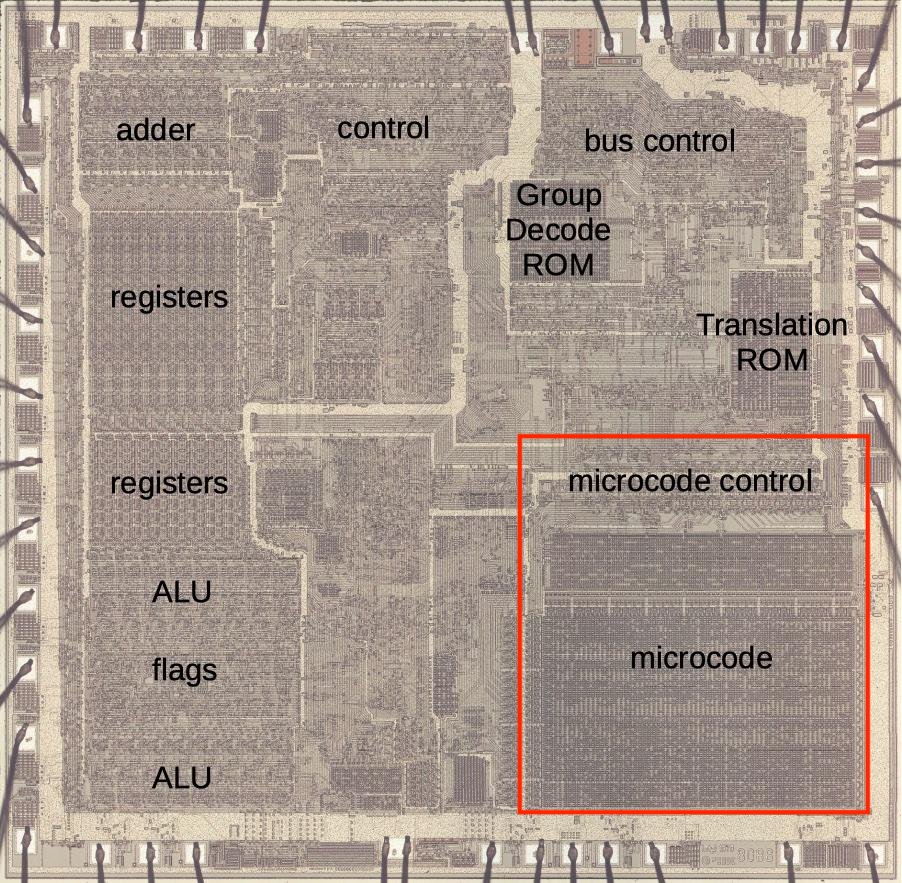This detailed diagram appears to be a blueprint or schematic of a microchip or computer motherboard. The entire image is primarily gray, with certain sections marked in darker shades and delineated by borders resembling those of a spiral notebook.

Starting from the left-hand side:
- The sections are labeled in sequence: "Adder," with "Registers" directly below it, followed by another "Registers" section.
- Adjacent to these on the right, we have two "ALU" sections, interspersed with a "Flags" section between them.
- Moving further to the right, the next section is the "Control" area.
- To the immediate right of this is "Group Decode ROM", set against a darker gray background.
- Above this and to the right, there's the "Bus Control" section.
- Below "Bus Control," situated to the right, is the "Translation ROM."

On the bottom right corner of the image, there is a conspicuous area bordered in red which contains a gray interior. Within this red-edged box, the text "Microcode Control" is prominently displayed, with "Microcode" written below it. 

The overall layout of the diagram gives an impression of meticulous organizational structuring, befitting a detailed depiction of microchip architecture or motherboard features.